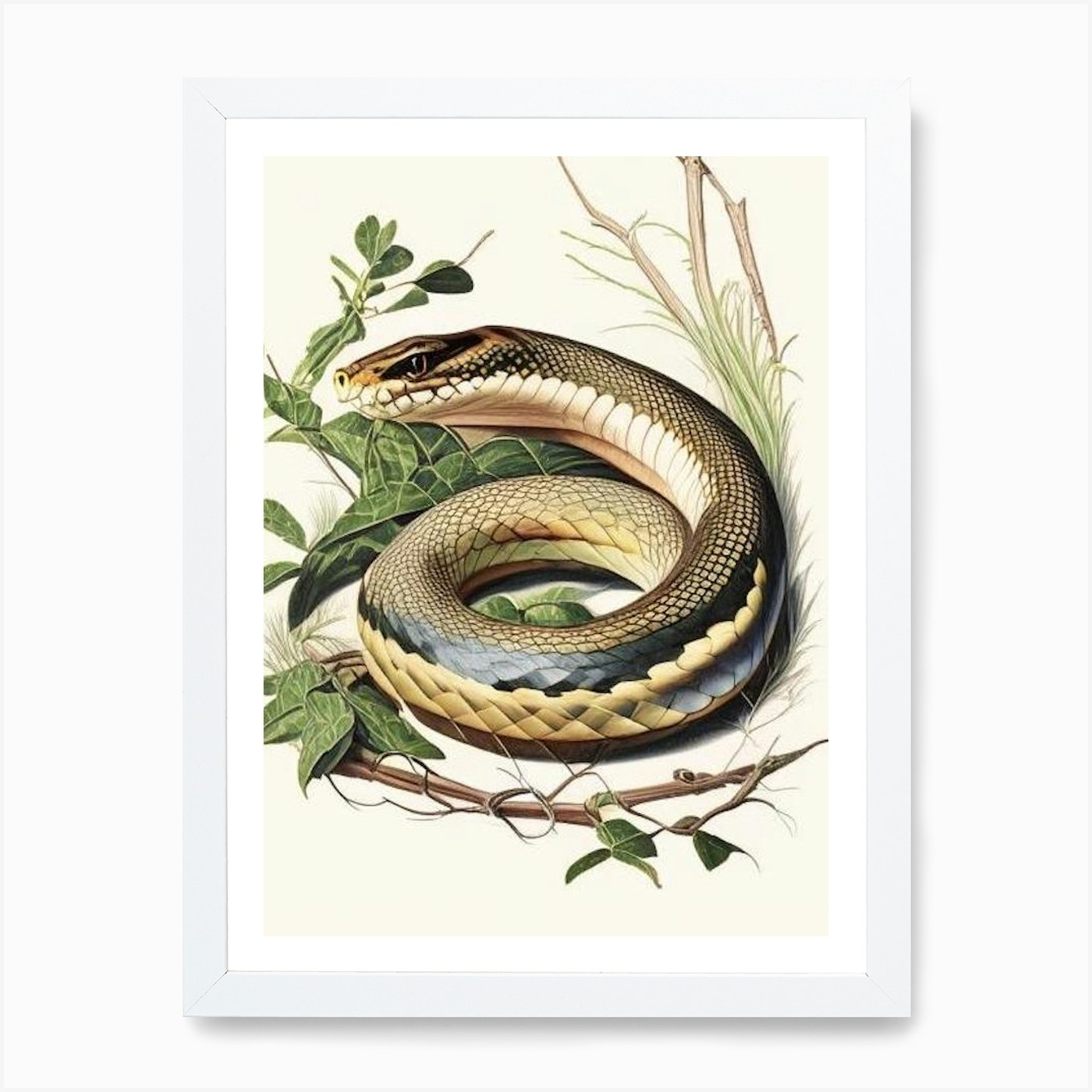The framed picture captures a detailed drawing of a gold or yellow-colored snake with a black diamond pattern running the length of its body. The snake is coiled and resting amidst thick, dark green leaves and vegetation. Its head is slightly raised, giving it an attentive look as if it is observing something nearby. Surrounding the snake are various elements of nature: a branch resembling barbed wire due to its intricate weaving, sparse green leaves, and grass-like textures above. Only one of the snake's eyes and its flaring nostrils are visible, further emphasizing its alertness. The overall scene suggests a cautious and potentially predatory stance, as if the snake is waiting for an unsuspecting passerby.